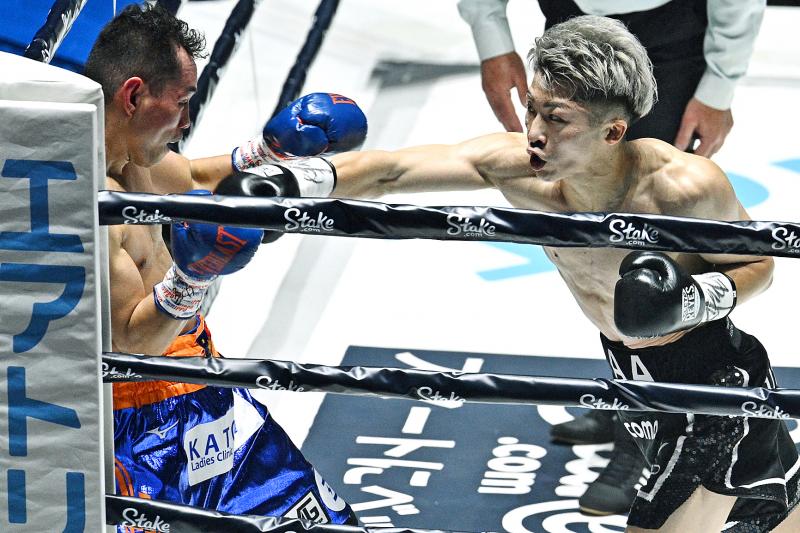This is a detailed photograph of an intense boxing match, seemingly set in Asia due to the presence of Asian characters in the advertisements around the ring. The focal point of the image is the action between two boxers. The boxer on the right, who appears to have frosted gray-blond hair cut very short around the ears, is wearing black boxing gloves and black shorts with "AA" and white designs on them. He is in the middle of delivering a powerful punch. His opponent, positioned against the ropes on the left side, has short black hair and wears blue and red shorts. He has blue and red Everlast boxing gloves raised defensively. The black ropes of the boxing ring feature the word "Steak" written in spaced-out white letters. The corner of the ring is padded in white with blue lettering that seems to be in an Asian script, and visible in the background, behind the aggressive puncher, is the referee observing the match intently. An advertisement written in Asian characters can also be seen in the corner of the ring.